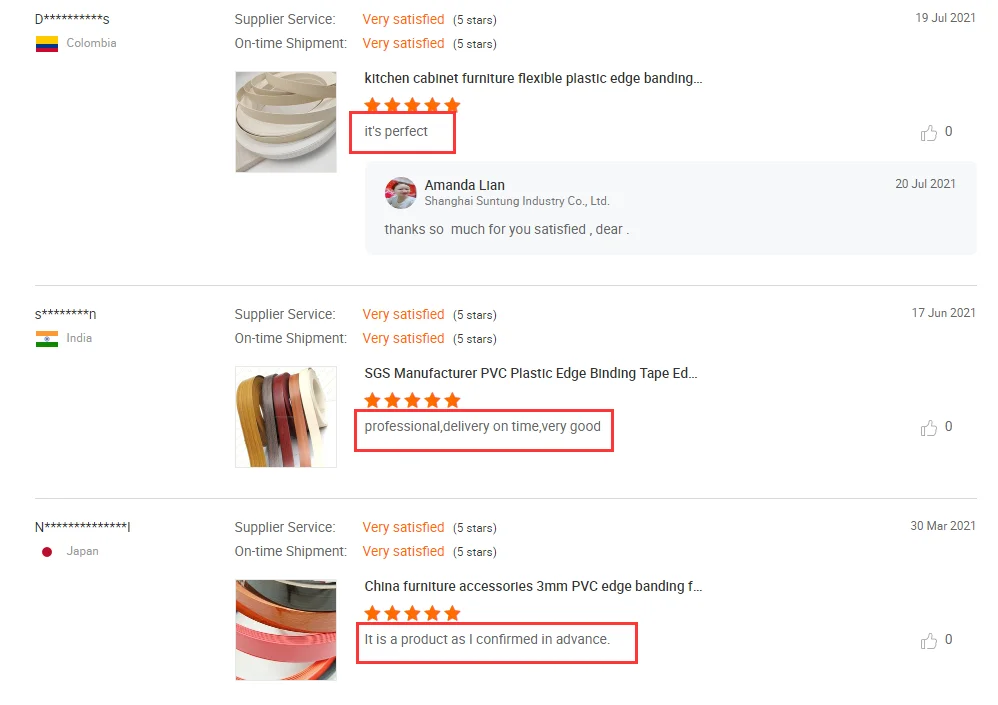The image features three separate reviews for PVC edge banding products, each from a different country. 

On the left side of the image, there is a small square icon of the Colombian flag, depicted with three horizontal stripes in yellow, blue, and red. Beside it is the word "Colombia." Below, there's a review indicating "Supplier Service: Very Satisfied (★★★★★)" and "On-Time Shipment: Very Satisfied (★★★★★)." At the center of this section, there's a small square image of plastic band pieces along with a five-star rating encased in a red rectangle proclaiming the product as "Perfect."

In the middle of the image, there is a flag of India marked by horizontal stripes of orange, white, and green. The review includes a "Very Satisfied (★★★★★)" rating. To the left of this section, more plastic edge binding tape is displayed in yellow, gray, red, pink, and white. A red outlined square indicates "Professional Delivery: On Time, Very Good."

The third review, on the right side of the image, features the flag of Japan, symbolized by a simple red circle. The review states "Supplier and On-Time: Very Satisfied (★★★★★)." More PVC edge banding in gray, orange, white, and pink colors is shown, accompanied by a five-out-of-five stars rating in orange. Lastly, within a red square, there's confirmation that the product was exactly as expected.

Overall, each review expresses high satisfaction with the supplier service, shipment timeliness, and product quality across various countries, as visually represented by their respective flags and the colored edge banding tapes.